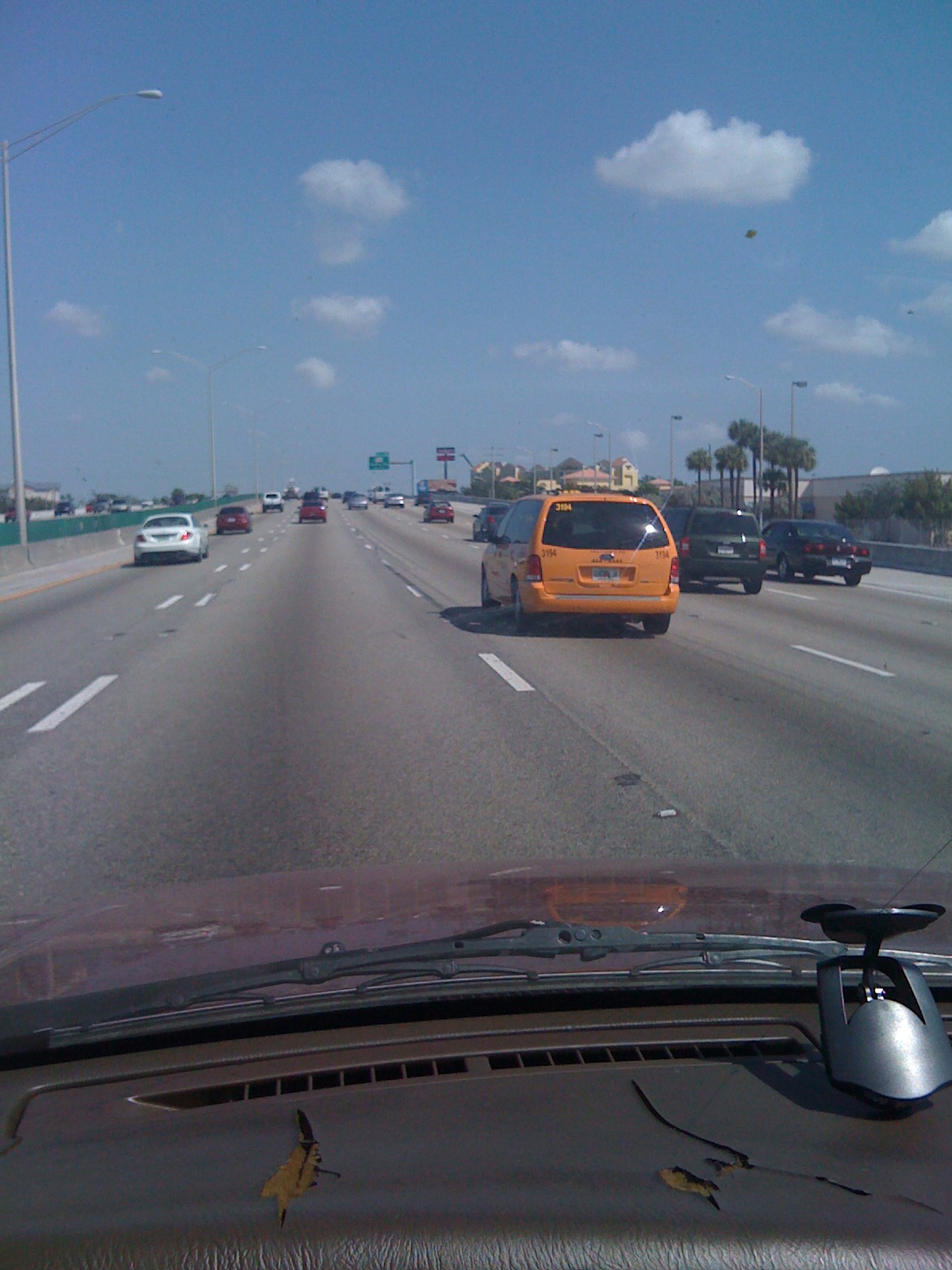The photograph appears to be taken from inside a car driving on a busy highway. Numerous vehicles populate the road, including a yellow van, a white car, and a dark green SUV, among others. The scene is framed by several palm trees that line the sides of the highway. The sky is a soft medium blue, dotted with small, fluffy white clouds. To the side of the highway, buildings are visible, possibly indicating a commercial area like a shopping mall. In the distance, a green highway sign can be seen, although the text on it is not legible.